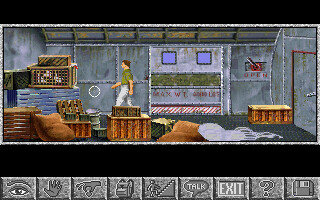The image is a screen capture from a vintage point-and-click adventure game, likely from the mid-1990s. The scene shows a man dressed in a green top and white pants standing inside a metallic, tubular room with a mechanical theme. The room is filled with wooden crates, one of which is painted blue, and burlap sacks. A large, open double door is visible, suggesting the possibility of moving to an adjoining area. There's also a garage-style door and a lever labeled "open," hinting at interactive gameplay elements.

At the bottom of the screen, a set of icons provides various control options, including an eye, a hand, a hand picking up objects, a backpack, stairs with a stick figure ascending, a speech bubble for talk, an exit sign, a question mark for help, and a floppy disk for saving progress. The cursor is represented as a white circle. The game's graphics, though dated, evoke a nostalgic feel reminiscent of 1990s computer games.